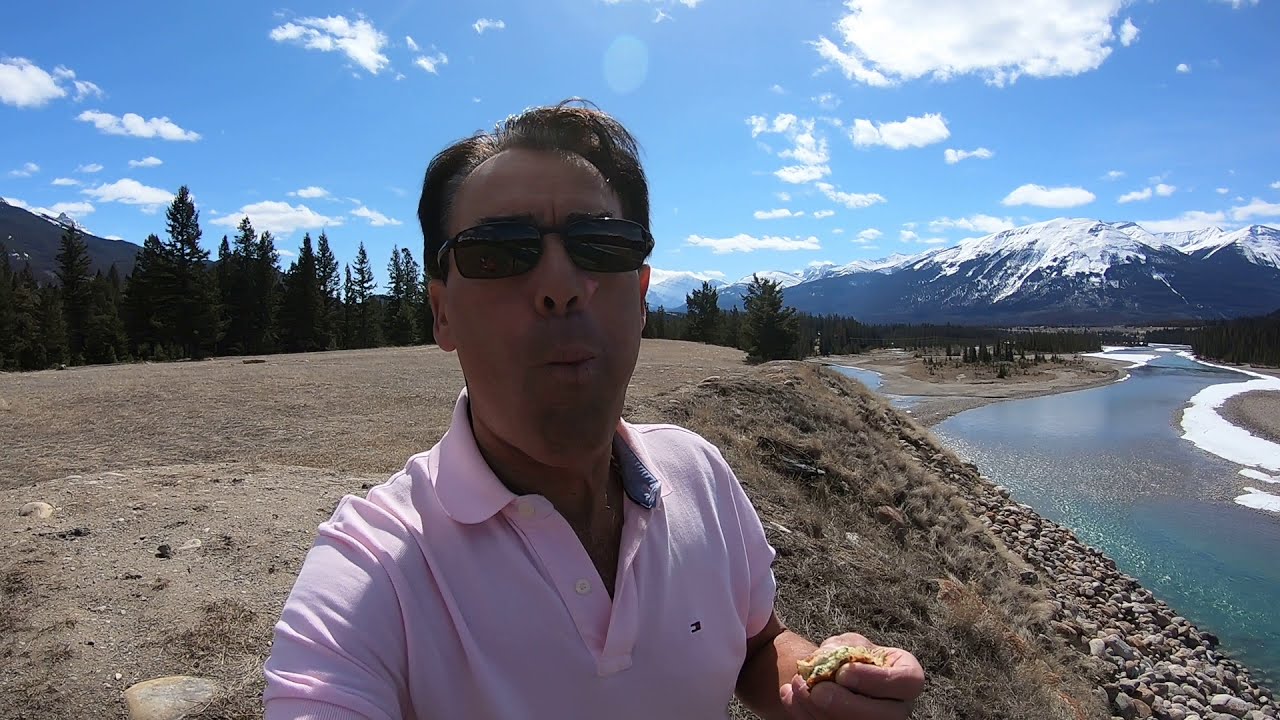In the selfie, a man wearing black sunglasses and a pink polo shirt with a gray inner collar stands in a natural outdoor setting. He is mid-bite into a pastry held in his left hand. The background showcases a dirt flat area leading to a dense collection of trees. To the right, a dark blue river with a rocky shore flows, its opposite bank dotted with snow. In the distant right corner, majestic mountains with snowy peaks rise against a light blue sky streaked with white clouds. The bright sky is also reflected in the man's sunglasses, adding to the vibrancy of this serene landscape.